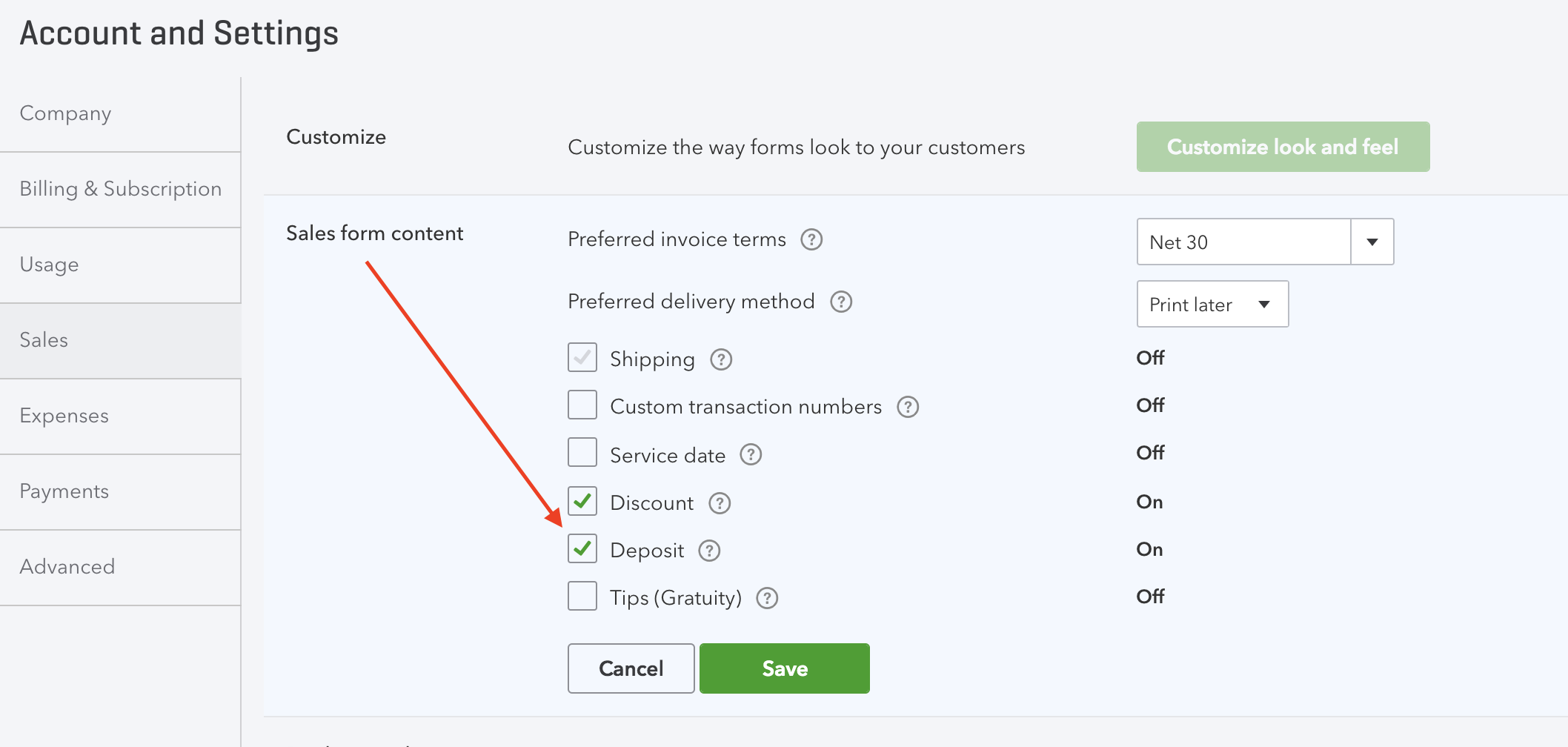This image depicts an 'Account and Settings' page set against a gray background. At the top left corner, the title "Account and Settings" is prominently displayed in bold black lettering. The main content is organized into a two-column layout. On the left side, a vertical navigation menu lists categories: Company, Billing and Subscription, Usage, Sales, Expenses, Payments, and Advanced. The 'Sales' category is slightly highlighted, indicating it is currently active.

On the right side of the menu, there is a customization section with the heading "Customize." Below this, it states, "Customize the way forms look to your customers." A green button labeled "Customize Look and Feel" in white text is prominently displayed.

Adjacent to the highlighted 'Sales' category, a blue-shaded box labeled "Sales Form Content" appears in the upper left corner. This box features a red arrow pointing downward towards the "Discount" and "Deposit" options. Parallel to this, an adjacent list specifies various settings including:

- Preferred Invoice Terms: Net 30 (with a dropdown menu)
- Preferred Delivery Method: Print Later (with a dropdown menu)
- Several checkbox options, including:
  - Shipping (checked)
  - Custom Transaction Numbers (checked)
  - Service Date (checked)
  - Discount (checked)
  - Deposit (checked)
  - Tips and Gratuity (checked)

At the bottom of this section, 'Cancel' and 'Save' buttons are available for user actions.